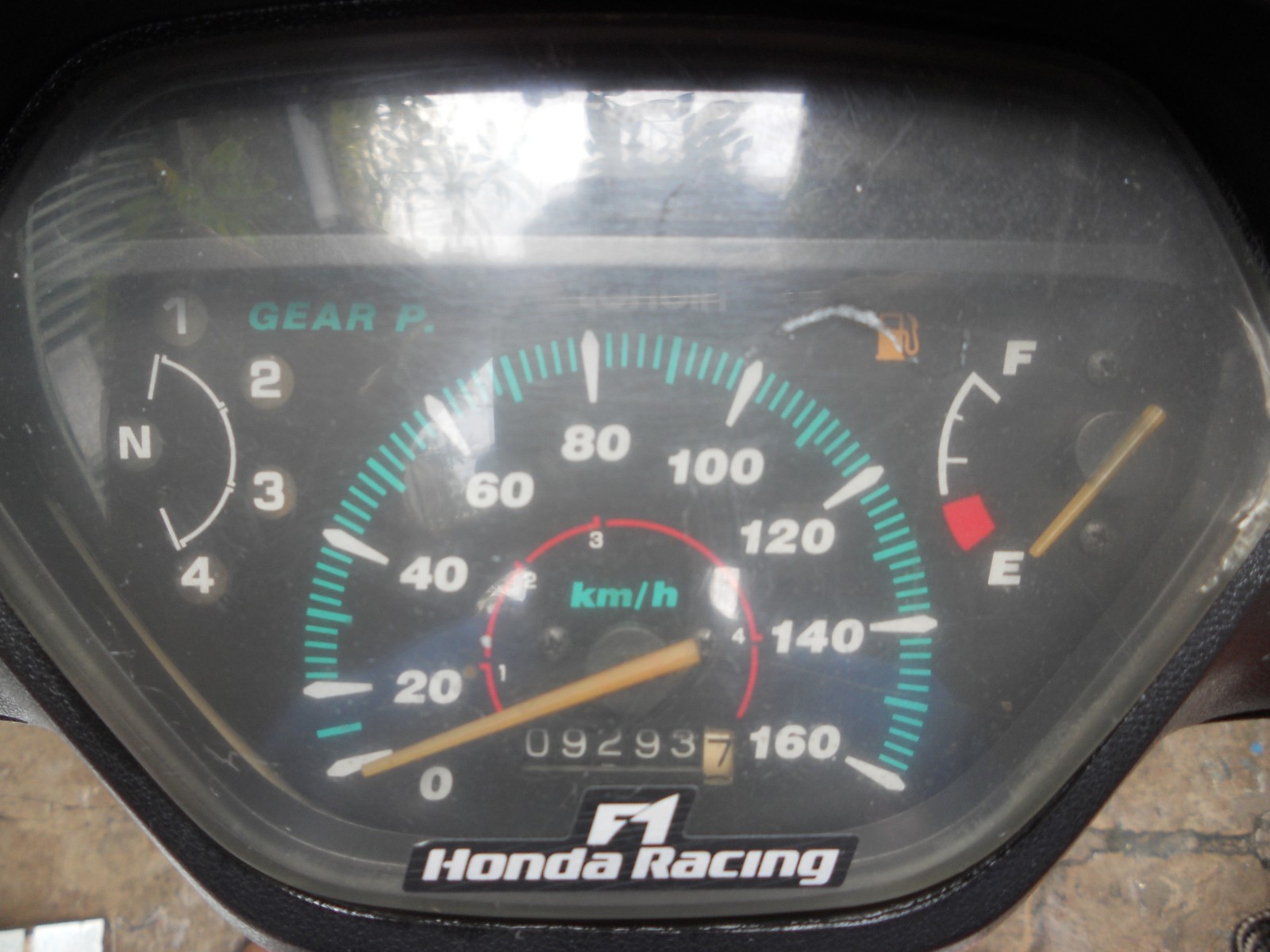The photograph captures the intricate details of a motorcycle's gauge cluster against a backdrop of brown bricks. Central to the image is the primary gauge, which prominently displays speed in kilometers per hour (KPH). This speedometer is marked with white increments of 20 KPH, from 0 to a higher maximum, and features a pale yellow needle. Within the central gauge, a smaller red subsection is marked with the numbers 1 through 4, evenly spaced apart.

Beneath the speedometer, the odometer reads 92,937, with the final digit distinctively highlighted in black on a white background. To the left of the cluster, a green indicator light displays the letter "P" overlaid on the word "gear," accompanied by another gauge arranged in a semicircular layout with numbers 1 through 4, and a central "N" for neutral.

On the top right corner of the speedometer, a yellow icon resembling a fuel pump indicates the fuel status. Adjacent to this icon is the fuel gauge, marked with an 'F' at the top for Full, an 'E' at the bottom for Empty, and a red square denoting the lower end of the spectrum. This gauge also utilizes a yellow needle. Reflecting off the gauge's protective glass or plastic cover is the white sky above, adding a subtle additional layer to the composition.